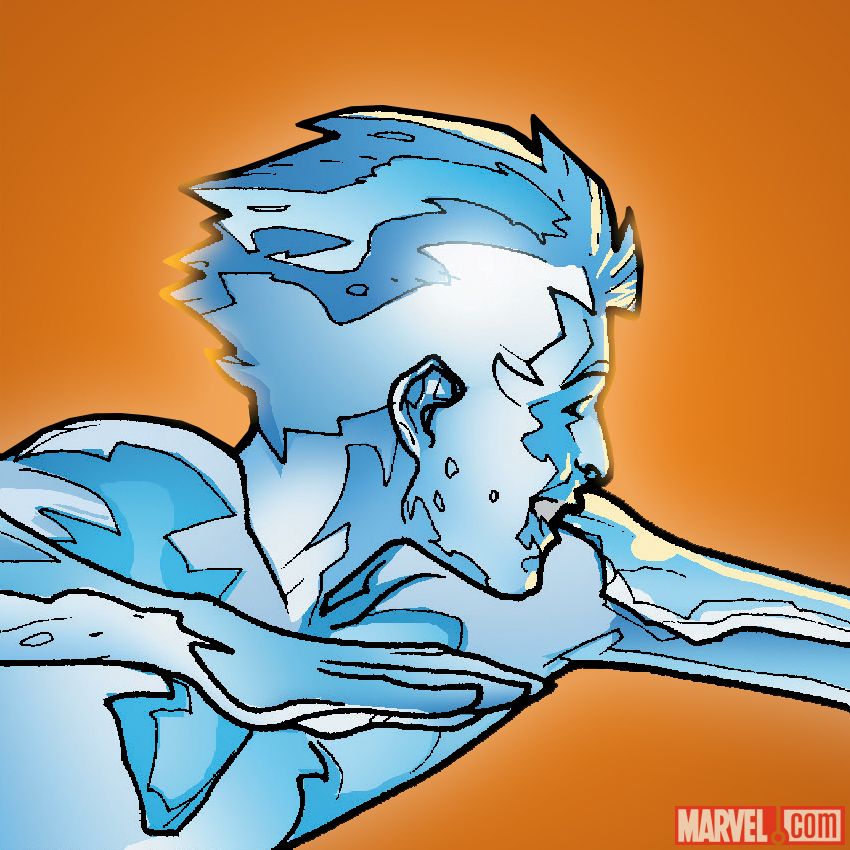This detailed computer-generated image features the Marvel character Iceman. The background showcases a gradient orange filter that transitions towards a burnt orange hue. Iceman is depicted in an action pose as if sliding, captured from his side profile. He has short hair and his figure is composed of various shades of blue and white, creating the illusion of being made out of ice. His arm is outstretched in front of him in a slicing motion, with the hand partially cut off by the frame, while the other arm is cocked back by his chin. The whole image is approximately 8 inches by 8 inches and rendered with lower to medium quality, likely using an online drawing tool or a paint program. At the bottom right corner of the image, the Marvel.com logo is prominently displayed. All elements in the image appear upright.